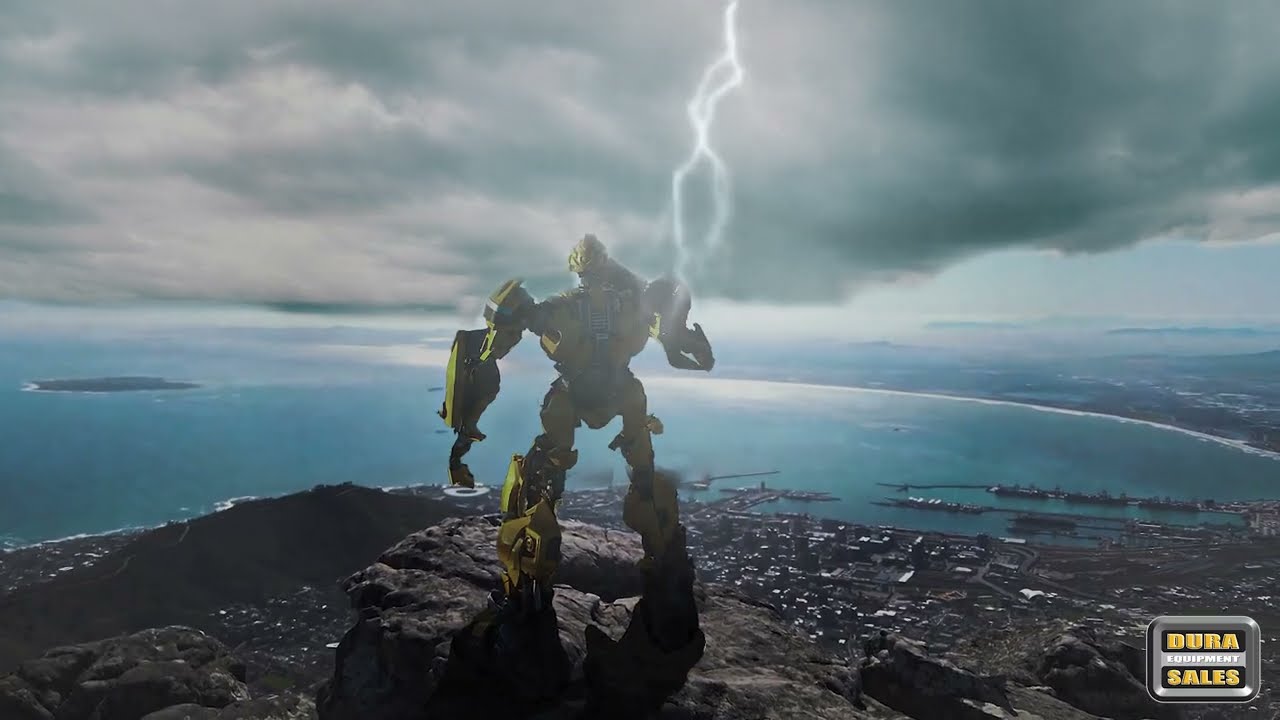This CGI image depicts a dramatic scene of a transforming yellow and silver robot, potentially resembling Bumblebee from the Transformers series, standing atop a cliffside. In the center of the image, a white lightning bolt dramatically strikes the robot. The scene offers a high vantage point overlooking a sprawling port city comprised of mostly rectangular, gray buildings. To the left, another mountain rises up, while the right-hand side reveals the shoreline of a vast blue body of water and white sandy beaches in the distance. Several cargo ships are docked in the harbor below. The sky is dark gray and stormy, but sunlight attempts to break through the ominous clouds, adding to the dramatic atmosphere. The intricate details of the cityscape, the stormy sky, and the striking robot contribute to the powerful visual impact of this scene.